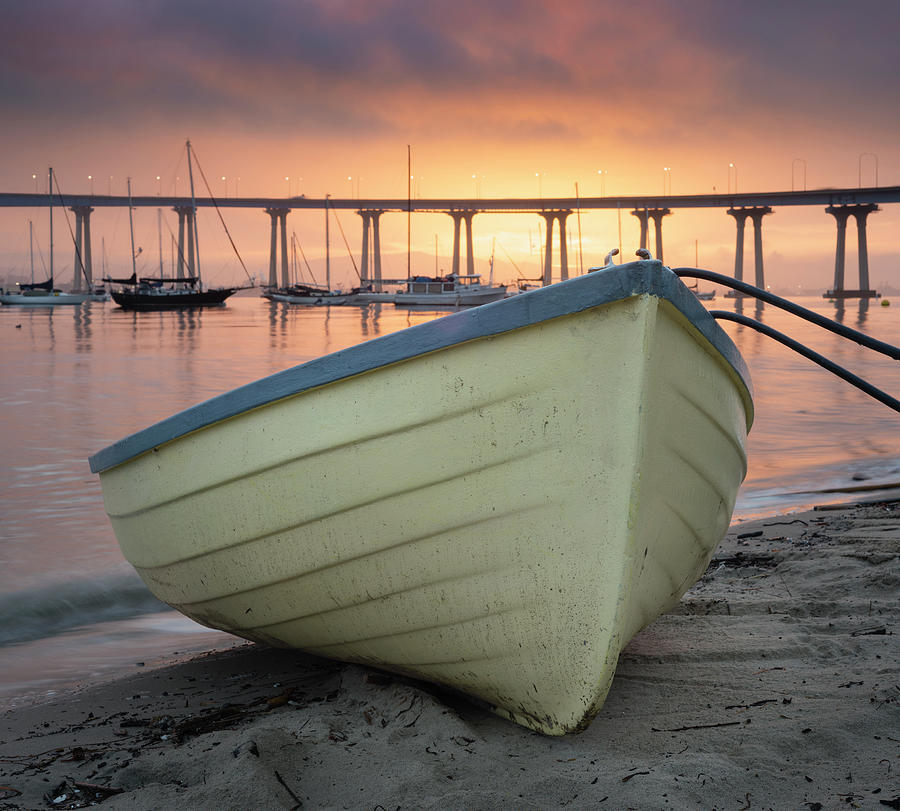This outdoor photograph captures the serene beauty of a sunset scene by the water. In the background, the sky is bathed in stunning hues of orange, pink, and yellow, accentuated by scattered gray clouds, indicative of a setting sun. Below the radiant sky lies a shimmering body of water reflecting these colors. Traversing the water is a modern bridge-like structure supported by several evenly spaced concrete pillars. Directly in front, several sailboats, with sails down, are lined up in a neat row, alongside some other boats including a pontoon or houseboat, giving the impression of a busy dock or port.

In the lower right foreground, detailed and prominent, a gray sandy beach meets the water. Resting on this sand is a small canoe-like boat; its base is a yellowish hue while the top edge features a contrasting gray border. The boat shows signs of wear and sand from being pulled onto the shore. This meticulous composition balances the ruggedness of the beach and boat with the calm and structured elements of the bridge and orderly boats, all under the warm twilight sky.